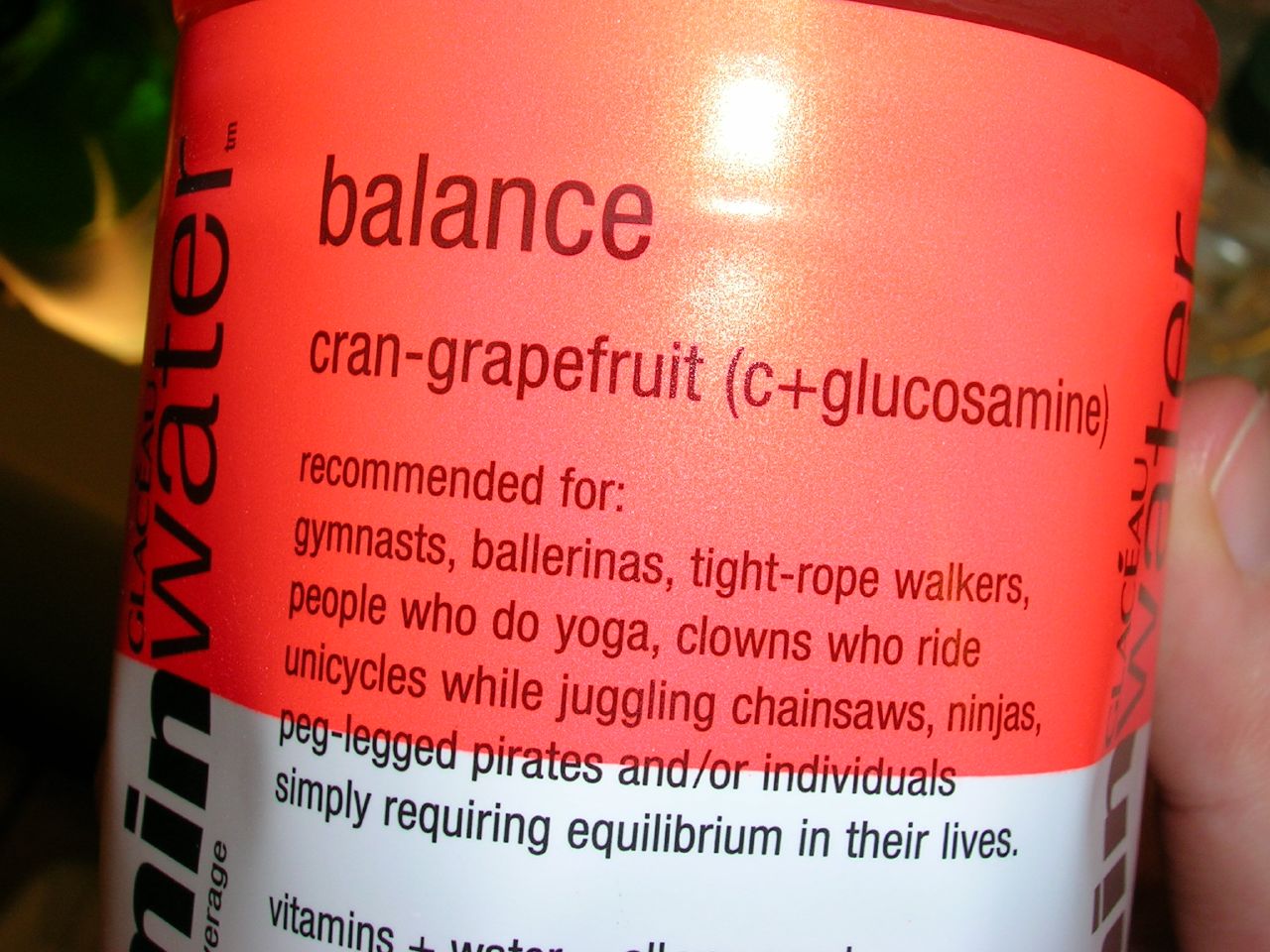This image captures a close-up of a vitamin water bottle label, prominently featuring a hand holding the bottle on the right side. The label is divided into a bright pinkish-red band at the top and a white section below it. The main black text at the top reads "Balance," followed by the flavor "Cran-Grape-Fruit" and in parentheses "(C+Glucosamine)." The detailed and whimsical text below recommends the drink for various acrobatic and balanced individuals, including "gymnasts, ballerinas, tightrope walkers, people who do yoga, clowns who ride unicycles while juggling chainsaws, ninjas, peg-legged pirates, and individuals simply requiring equilibrium in their lives." The left side of the image shows partial lettering of "MIM" and "water" vertically, and the bottom part of the white label is partially obscured, cutting off the text.